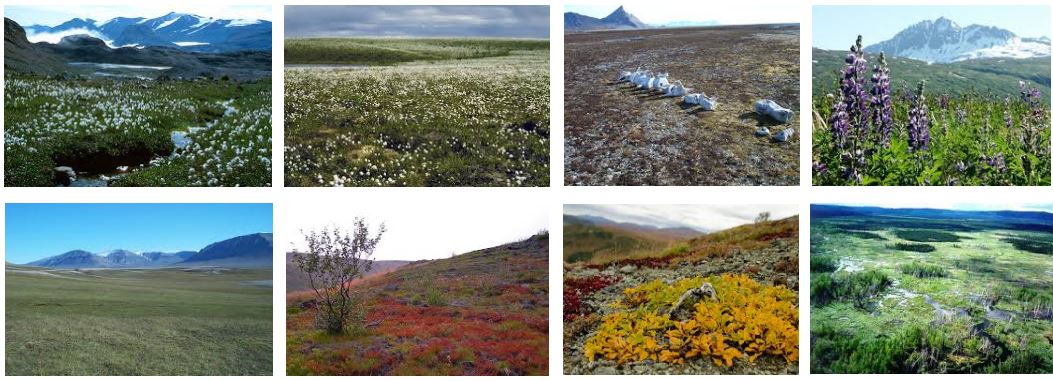The image features a rectangular array of eight small outdoor photographs, all separated by thin white strips. The photographs are arranged in two rows of four. The top left photograph captures a stunning mountain range in the background with a small brook and tall green grass dotted with white flowers in the foreground. Moving to the right, the second image showcases a cloudy gray and white sky above a field dominated by green grass and white wildflowers. The third photo features a flat expanse of land, possibly the top of a mountain, with something indistinguishable, perhaps ducks, in the center. The upper right image presents a beautiful snow-capped mountain in the background, with tall green grass and purple flowers, likely lupines, in the foreground. 

On the bottom row, the leftmost photograph portrays flat green land against a backdrop of mountains and a blue sky. The second image from the left on the bottom captures a small tree or bush to the left side, with reddish-purple grass and a cloudy white sky above. The third image on the bottom row shows a patch of yellow leaves in the foreground with mountains in the distance. The bottom right photograph provides an aerial view looking down at a landscape abundant with green and white elements.

Each photograph emphasizes the natural, uninhabited wilderness, highlighting various seasonal changes with hints of snow, fields of wildflowers, and diverse grass colors. The entire collection seems to depict a place possibly located in the American Northwest.